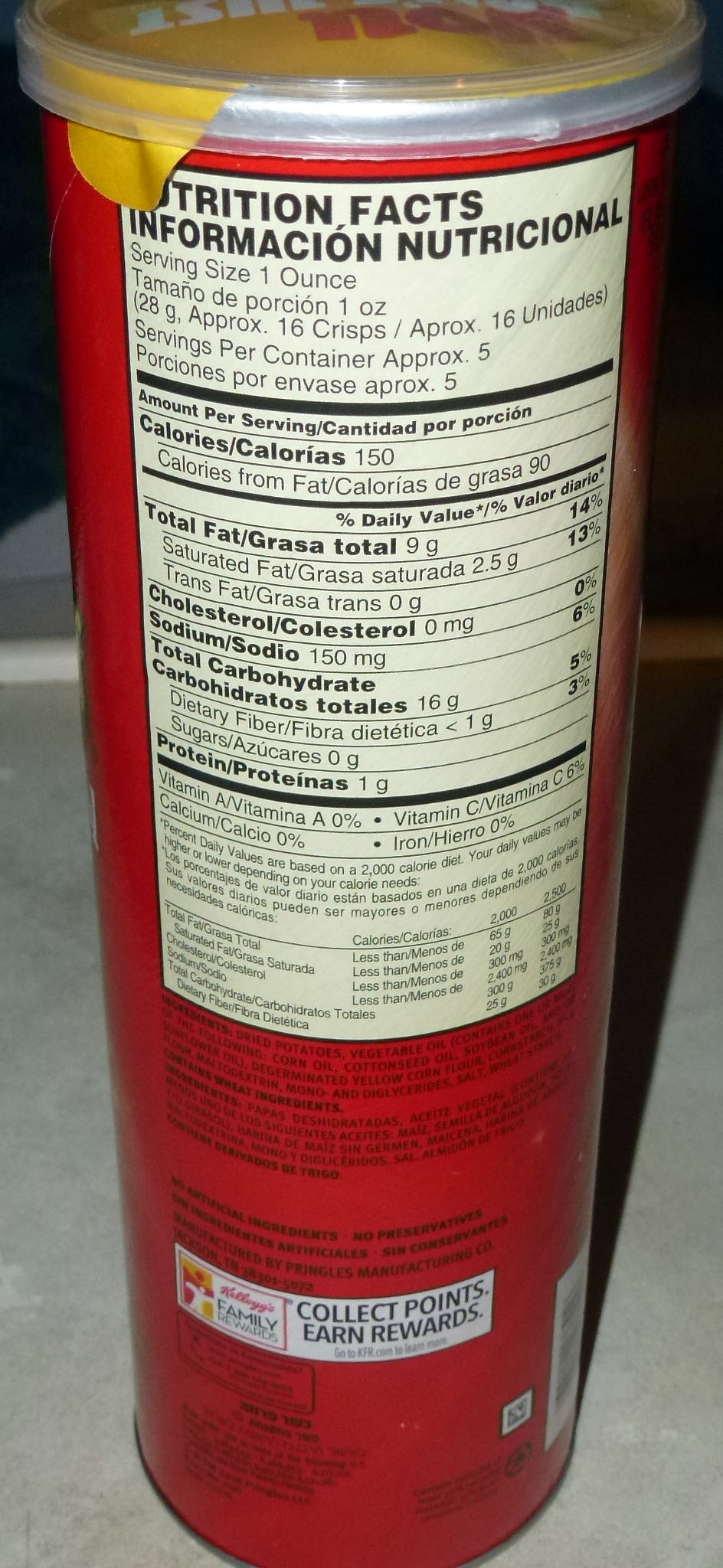This image displays the back of a red Pringles can, prominently featuring the Nutrition Facts panel. The panel indicates a serving size of one ounce, which equals approximately 16 crisps, and notes that there are roughly five servings per container. Each serving contains 150 calories, with a breakdown of 9 grams of total fat, zero cholesterol, 150 milligrams of sodium, 16 grams of total carbohydrates, less than one gram of dietary fiber, zero grams of sugars, and one gram of protein. Smaller text provides additional nutritional details, though these are not legible in the image. An additional label on the can advocates for Kellogg's family rewards program, encouraging consumers to collect points and earn rewards. The can is topped with a clear lid covered by a yellowish-orange seal, creating a contrast against the red can and the black and white nutritional information.